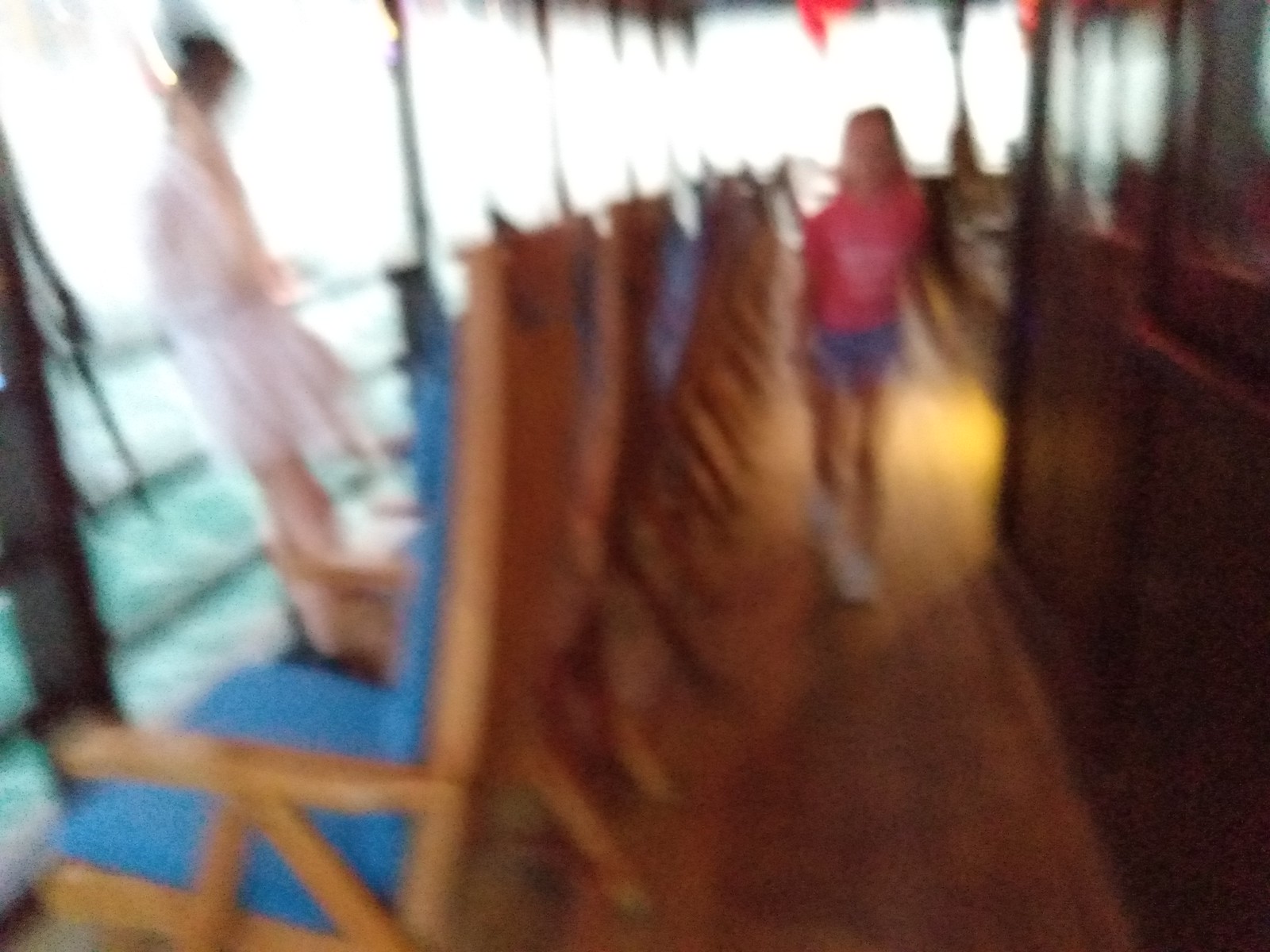This photo, taken aboard a boat, captures a scene on the deck despite its fuzzy quality. The deck, made of wood planks, stretches across the middle of the image. On the right, the center of the boat is barely visible. A person, likely a female, is walking along the deck; she is dressed in a pink t-shirt and blue shorts. To the left, wooden chairs are neatly arranged for passengers who wish to sit by the railing and gaze at the choppy ocean waters. Leaning against the rail, a woman in a flowing white dress is visible. Beyond her, the ocean stretches out, blending seamlessly into a bright, featureless white horizon.